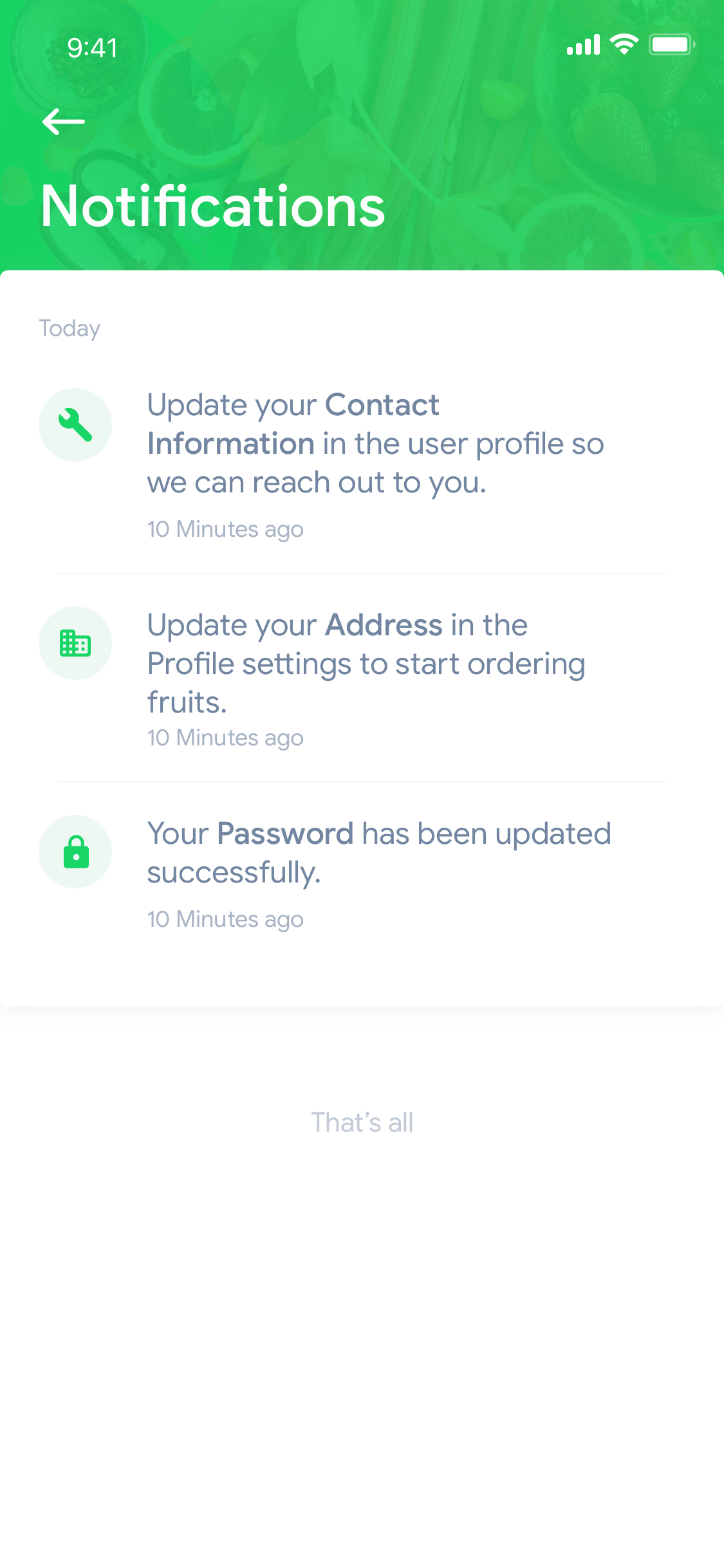This screenshot depicts a cropped view of an application running on a smartphone, possibly an older Android device, inferred by the design of the icons, although the absence of navigation buttons at the bottom leaves some ambiguity; it might alternatively be an older iOS device. At the very top, a textured banner stretches across the screen, displaying the word "Notifications" in white text along with a left-pointing arrow, also in white.

Below this banner, the background transitions to white and features three distinct items. These items are separated by thin, nearly imperceptible gray lines. Each item has a green icon to its left—first, a wrench icon, followed by an icon depicting a couple of lists, and lastly, a padlock icon.

Accompanying each icon, in descending order, black text details:
1. "Update your contact information and user profile so we can reach out to you."
2. "Update your address in the profile settings to start ordering fruits."
3. "Your password has been updated successfully."

All three notifications indicate they were received "10 minutes ago." At the bottom, the phrase "That's all" appears in very faded text, suggesting there are no additional notifications for today. The notifications displayed are generic updates pertinent to the app's usage.